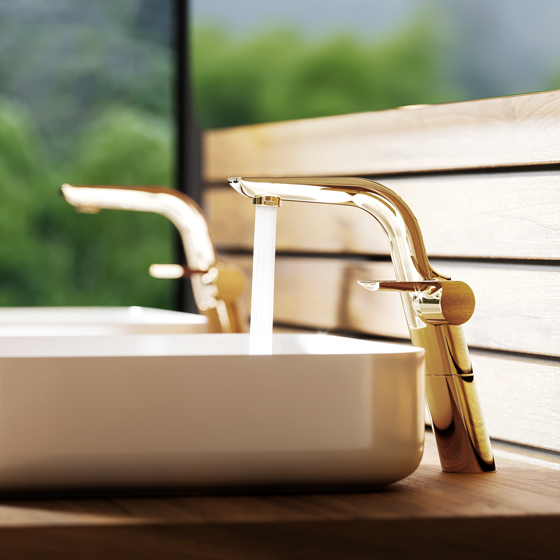In the image, there is a detailed close-up of a modern bathroom sink setup with a focus on the nearest sink. The scene features two side-by-side sinks, though the second one is noticeably blurred and out of focus. The prominent sink in the foreground has a sleek, shiny gold faucet with a single handle, which is currently turned on, allowing water to pour into a shallow, square-shaped, cream-colored basin that sits above the countertop. The rectangular basin rests upon a medium brown wooden countertop and is not embedded within it. Surrounding the sink area is a backsplash made up of four wooden panels. In the blurred background, a two-paned window reveals hints of outdoor greenery, adding to the serene ambiance. The overall composition highlights the contemporary design elements of the sink while subtly incorporating the natural scenery outside.